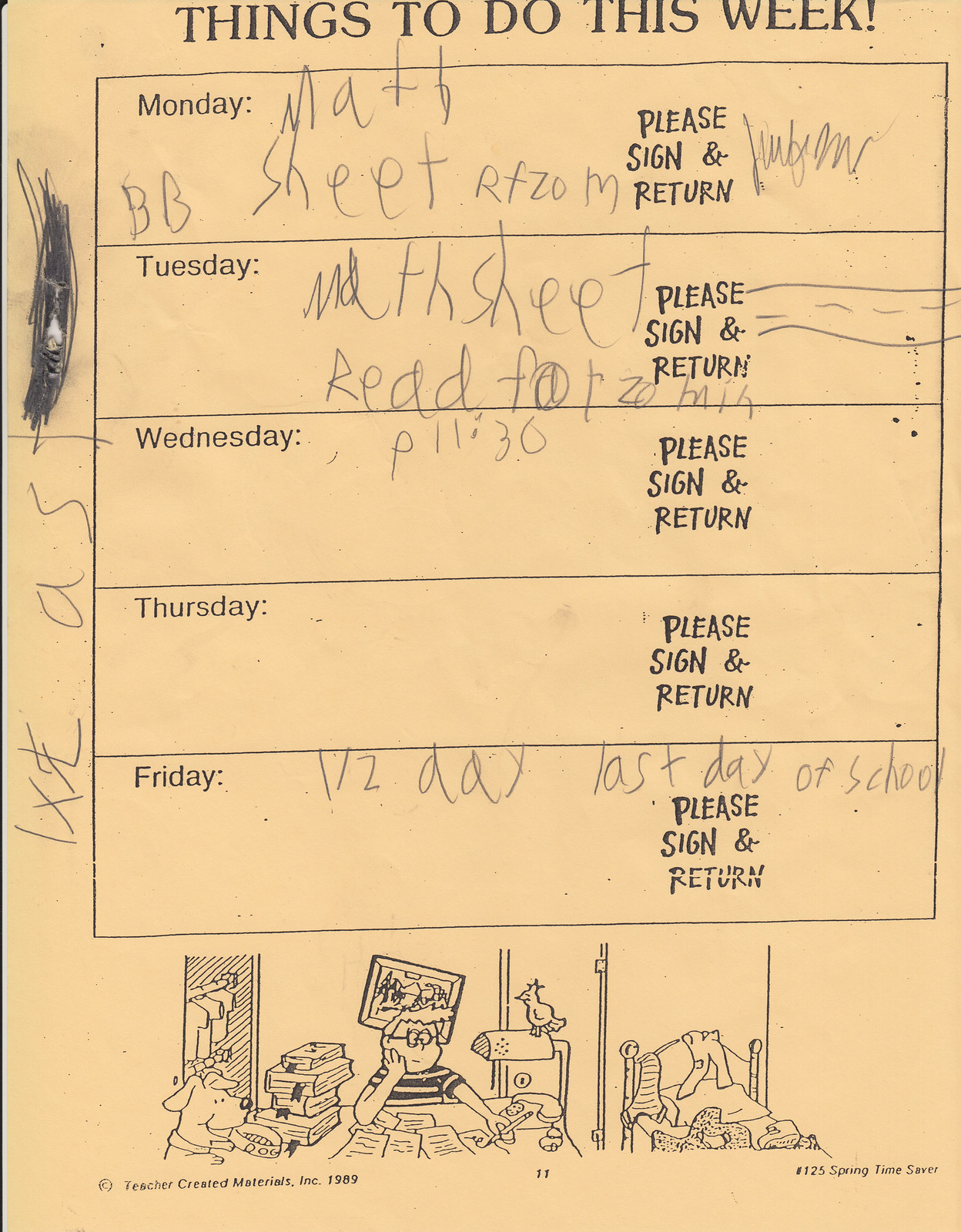This is a discolored, yellowed school worksheet titled "Things to Do This Week" at the top. The template has five outlined long rectangles labeled Monday through Friday on the left-hand side, each accompanied by "Please sign and return" on the right. At the bottom, there are cartoony drawings of a boy with small glasses seated at a desk with a pencil in his hand, a bird perched on a desk lamp to his right, a stack of books to his left, a dog holding a collar, and a messy bed with clothes strewn about. The worksheet is copyright Teacher Created Materials, Inc., dated around 1989 or 1981.

The student's handwritten entries, in large, clumsy writing, read: 

- Monday: "Math BB sheet RF ZOM" with a barely legible signature beside "Please sign and return."
- Tuesday: "Math sheet read for" followed by unreadable marks and some doodles next to "Please sign and return."
- Wednesday: "P11:30" appears beside "Please sign and return," with no signature.
- Thursday is blank except for "Please sign and return."
- Friday: "Half day last day of school" written above "Please sign and return."

Additional scribbles and doodles mark the left side of the sheet, including illegible writing that adds to the cluttered appearance, indicative of a young student's use.